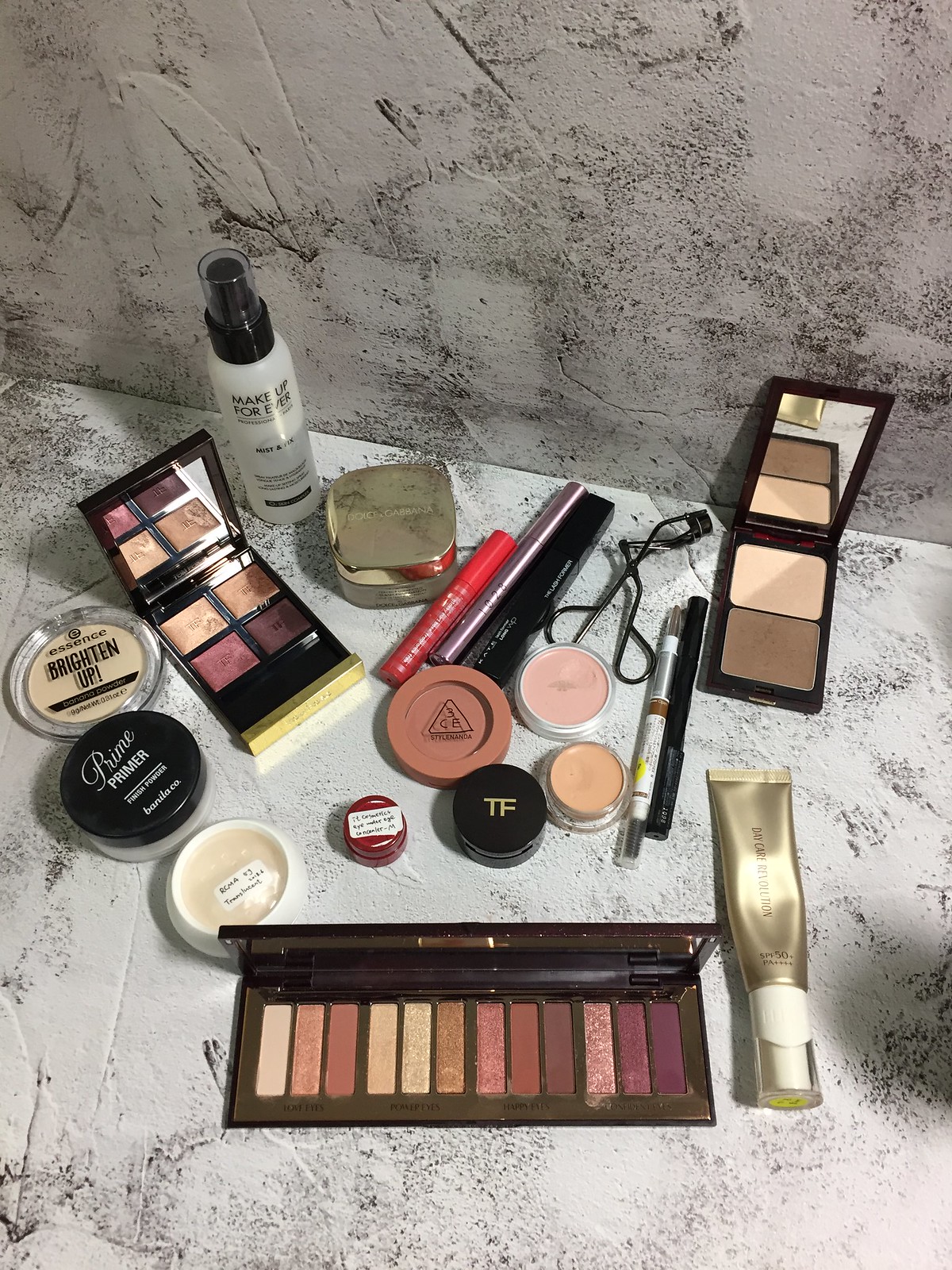This image is taken from a slightly elevated angle, giving a clear view of the scene below, while also including some of the background. The background appears to be the exterior of a structure, characterized by a light gray concrete wall marked with various dark gray and black smudges and lines, suggesting a rough texture with small bumps and cracks. This same concrete texture extends to the surface on which various makeup items are displayed.

The assortment of makeup products includes an open eyeshadow palette revealing multiple colors, a smaller quad eyeshadow palette also open to show four shades, a "Brighten Up" concealer, and a bottle of face spray. A contour palette is also open, displaying a mirror and dual shades for highlighting and contouring. Several other items are scattered around, such as mascara, eyeliner, and an eyelash curler. All products appear to be in pristine, unused condition, meticulously arranged on the concrete surface.